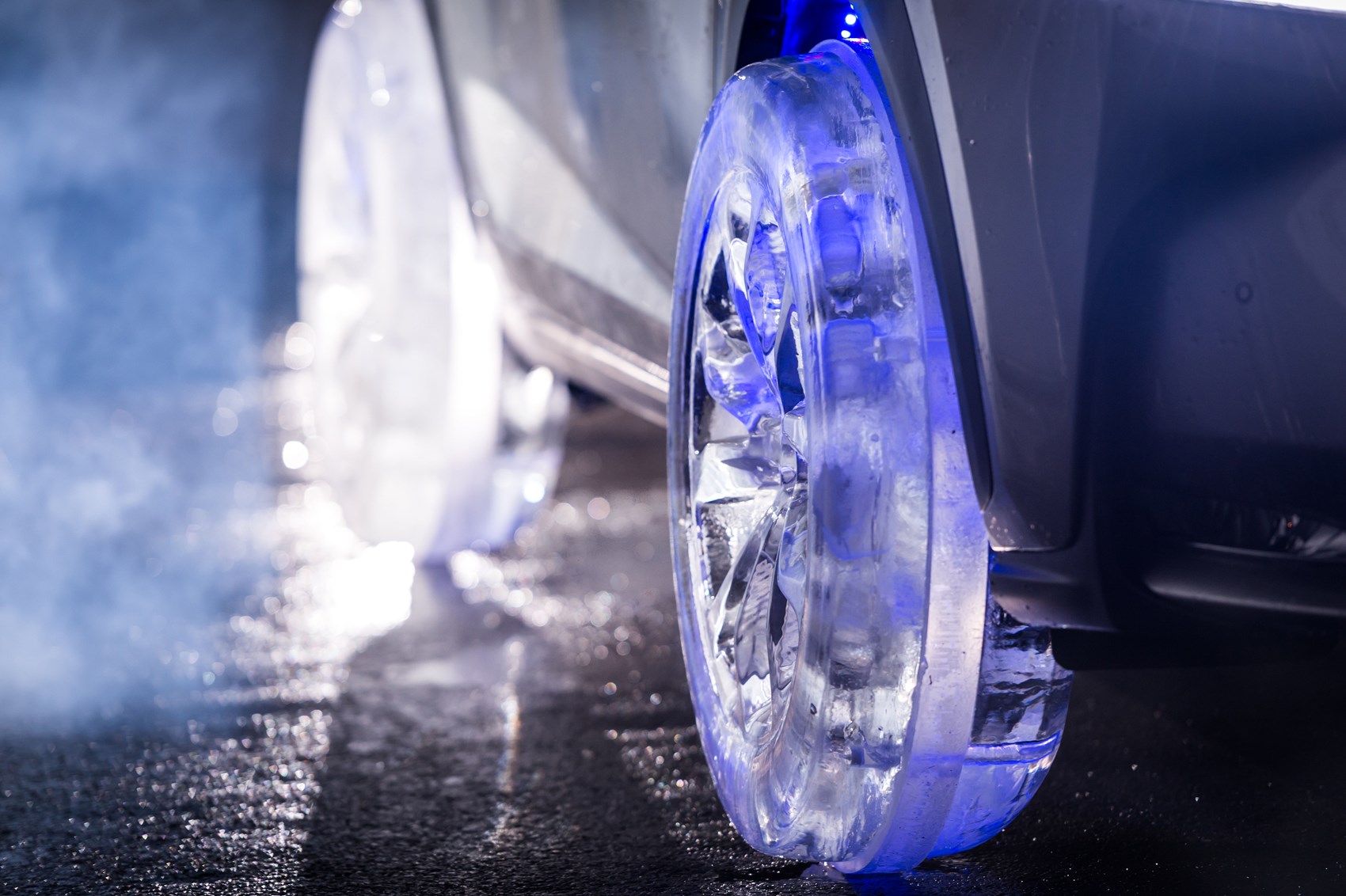This image captures the bottom right-hand portion of a modern, dark gray car at night, resting on black asphalt that appears wet, reflecting light. The focus is on the vehicle's tires, which astonishingly appear to be made entirely of ice. The front tire exhibits a translucent blue hue, likely due to a blue light shining on it, making it seem as though it is encased in blue ice. The rear tire, while also made of ice, lacks the blue illumination and instead shines a bright, pure white. The background reveals another tire, blurred yet discernibly white. Adding to the ethereal atmosphere is a cloud of white smoke or fog on the left side of the image, tinged with a faint blue reflection. The overall scene is both surreal and striking, with the luminous icy tires contrasting starkly against the dark, slick pavement.